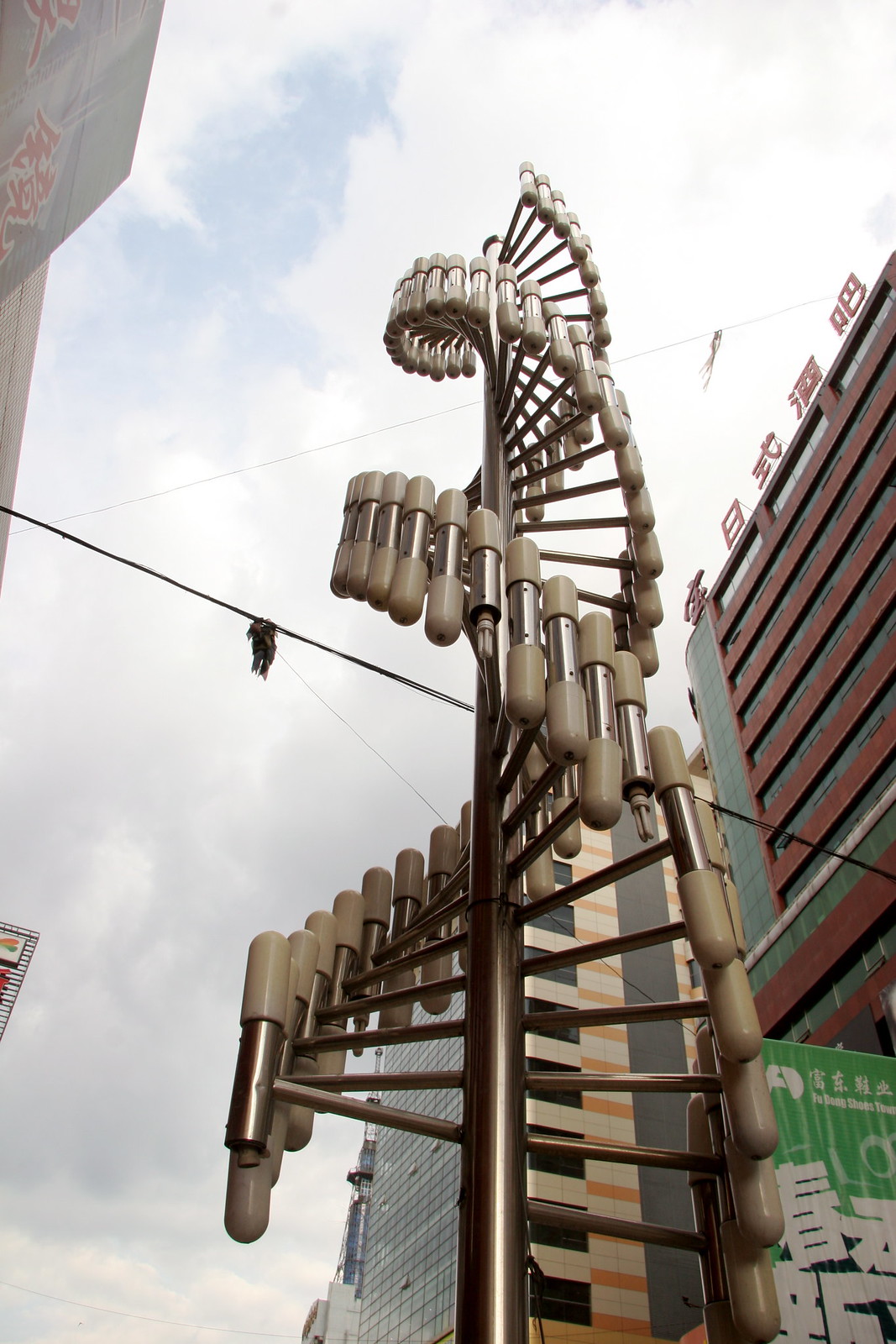The image depicts a large, intricate metal structure reminiscent of a spiral staircase or DNA helix, featuring a central brass-colored pole with multiple horizontal strands, each adorned with vertical oblong poles capped in white. This design creates a swirling, spiraling effect as it ascends into the air. The photograph is taken from a bottom-up perspective on an overcast day, with the sky appearing predominantly gray with patches of blue. To the right of the structure stands a sizable gray and red building, the top of which displays characters in either Chinese or Japanese. Behind the central structure lies another building characterized by its tan and orange hues, vertical black stripes, and multiple windows. Additionally, a green sign with white Asian characters is visible in the bottom right corner. Furthermore, a couple of cables are draped diagonally across the scene, intersecting from the upper left to the bottom right and from the upper right to the bottom left.